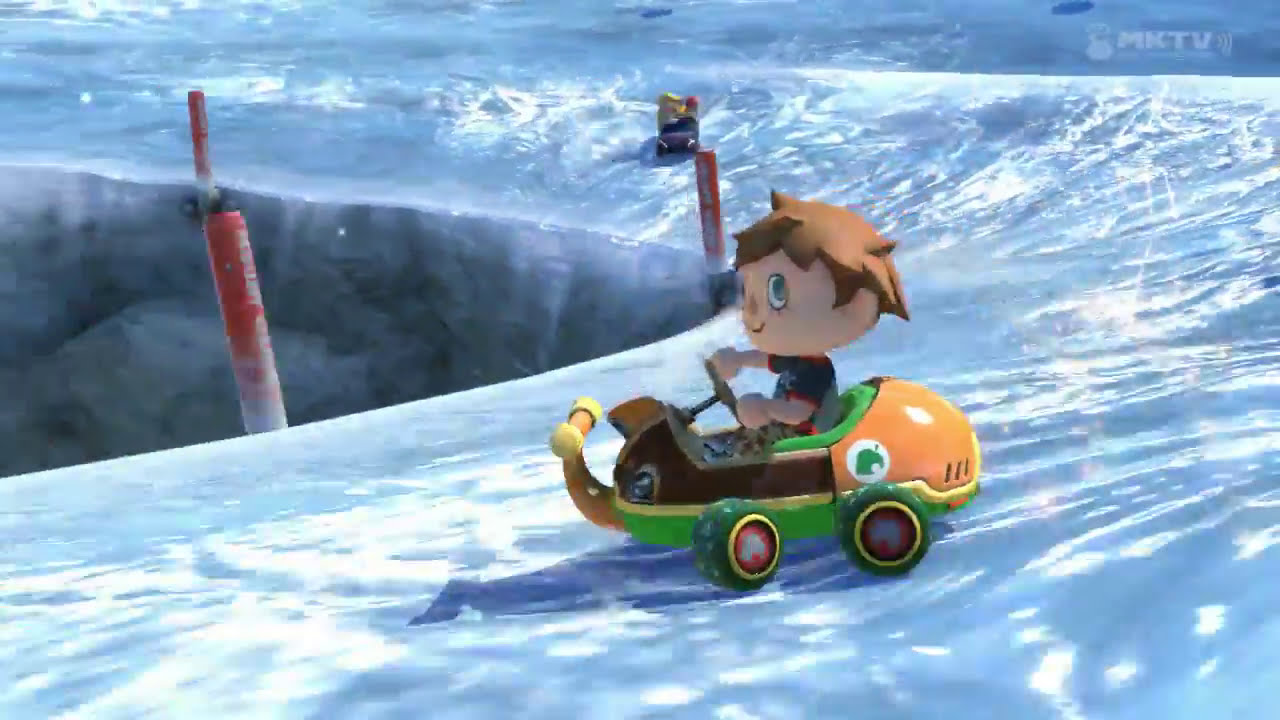This detailed computer-generated image showcases a scene resembling an animated children's TV show or movie, potentially similar to Mario Kart. The focal point is a cartoon boy with short brown hair, dressed in a t-shirt, riding a toy-like snowmobile car. The car is vividly colored with green as the primary hue, accented by a white and orange trim, brown details, and green wheels with a red rim. The boy appears to be navigating a snowy or icy track, perhaps a frozen dam or a perilous snow-covered hill with scattered red poles marking the course. A significant drop-off or hole dominates the middle of the image, suggesting a high-stakes race. Another car can be seen in the upper middle of the image, hinting at competition. The upper right corner of the scene prominently features "MKTV" in white lettering, indicating the source or branding of this thrilling, TV show-like environment.